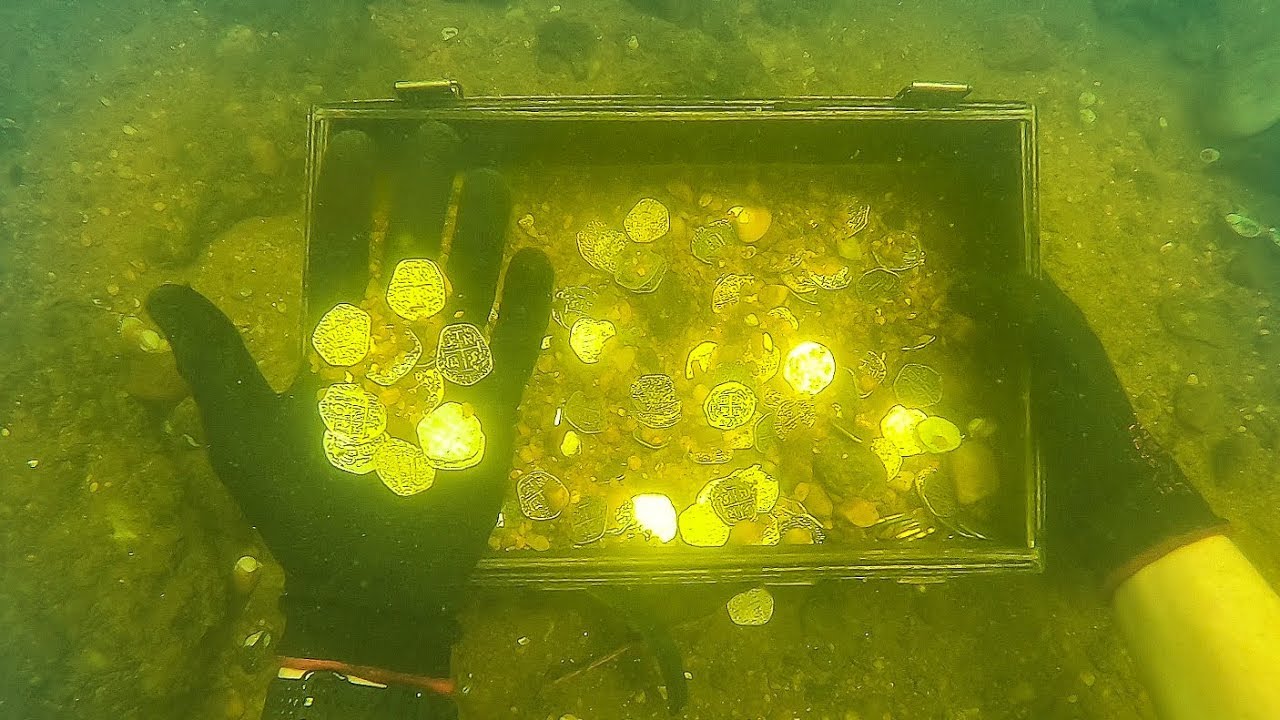The underwater image depicts a diver discovering a treasure chest filled with coins. The overall color palette is a yellowish-green, resembling mossy, dirty water. The diver is wearing black gloves, made from either rubber or a thin canvas material, and a diving watch is visible on the wrist, though its face is not shown. The diver’s right hand grips the box, while the left hand is turned upwards, displaying several oddly-shaped coins, which appear to be hexagonal with rounded edges, in various states of preservation—some gold, some brown, and possibly rusted. These coins shine amidst a seabed cluttered with rocks, dirt, and sand. One of the coins lies just behind the box on the ground, contributing to the scene's authenticity and age.